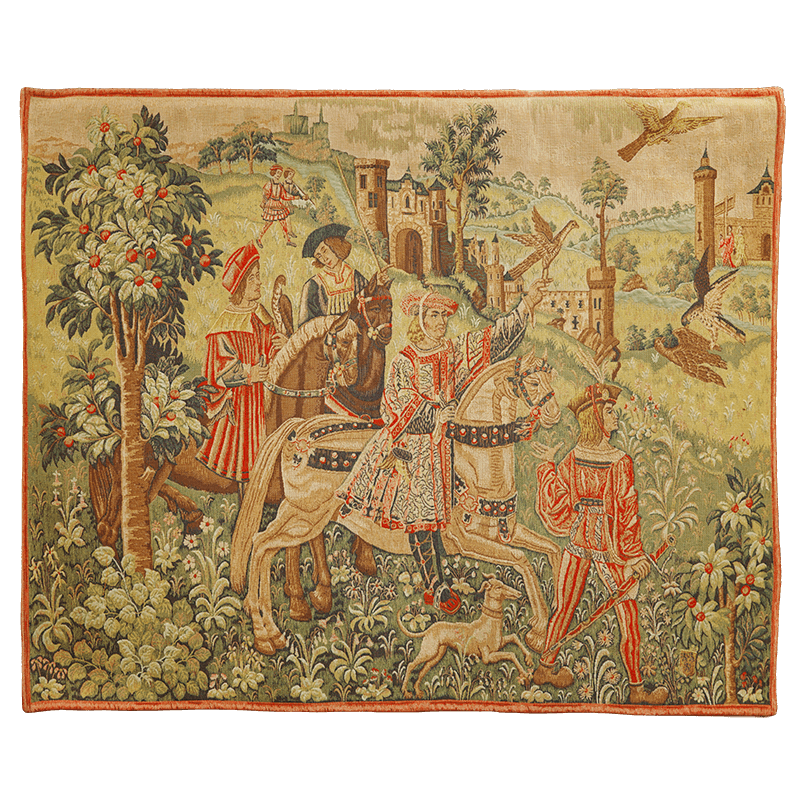The image depicts an intricate, aged tapestry showcasing a medieval scene with rich details and muted colors, primarily shades of brown, with red prominently featured. The vertical, rectangular tapestry is bordered by a dark brown trim, framing a vivid outdoor setting. The scene is populated by multiple figures, including three individuals riding horses: a dark brown, a light brown, and a beige horse. The central rider, a woman in a white dress with red trim over black pants, and a red hat secured under her chin, holds her hand up with a bird perched on her finger. Nearby, a man in a red outfit stands holding a sword, seemingly guiding the procession. Smaller details enrich the scene: a brown dog runs alongside, and several birds hover in the sky above. The backdrop reveals rolling hills dotted with medieval castles, each adorned with green-blue roofs. The lush setting is filled with vegetation, including trees with red berries and white flowers. The tapestry's composition evokes a timeless sense of a royal hunt, with a harmonious array of historical attire and a bustling, verdant landscape.